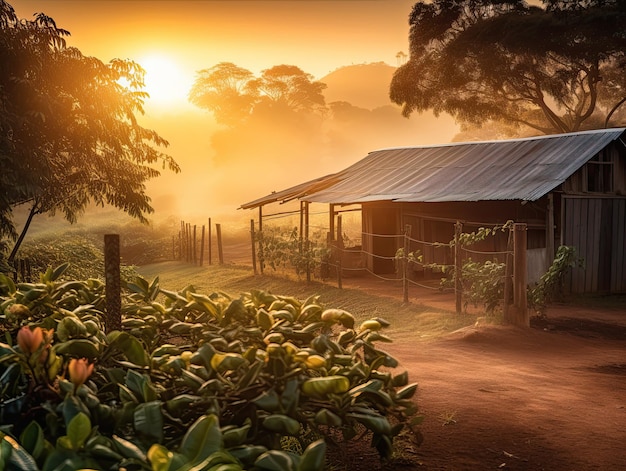The image presents a rural, rustic scene that appears to be at either sunrise or sunset, evident from the peach, orange, and brown hues in the sky. At the top center of the sky, the sun shines brightly with a white glow. Dominating the right side of the image is a shed with a gray roof, fronted by a twine fence made of wooden poles. Surrounding the shed and extending toward the left are lush plants with green leaves, some bearing pink flowers. The scene also features various trees; one tree is visible above the shed, while another stands to the left side, under which more plants and potential crops, possibly including peppers, are visible. The ground below the plants spans a range of colors from brown at the bottom to green in the center. The overall atmosphere of the image, which appears computer-generated or animated, captures the serene and climactic moment of either dawn or dusk in a charming farmhouse setting.